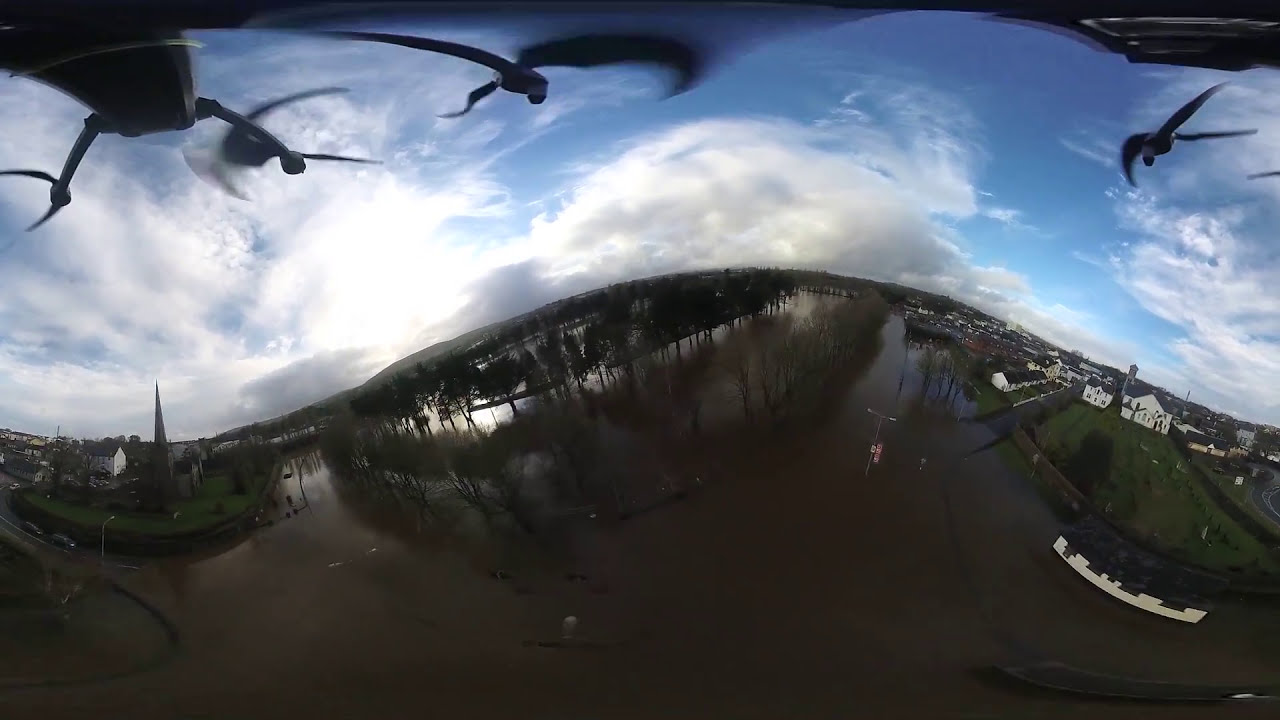This image captures a chaotic and distorted aerial view, likely taken from a helicopter or drone, showcasing a serene yet somewhat muddled landscape. The fish-eye lens distorts the scene, creating a sense of motion and surrealism. In the foreground, there's a large, brown river winding through the landscape, with a circle of trees situated centrally within the water's edge. A white boat is visible in the lower right corner, adjacent to a grassy patch.

The middle ground is dominated by a variety of natural and man-made elements. A cluster of trees forms a dense patch near the center, surrounded by muddy terrain, while scattered white buildings, possibly residential houses, make their presence known in the background. Some of these buildings include a church with a prominent steeple, and just to its left, a white house stands out. Numerous additional structures line the horizon, lending an impression of a nearby town or settlement.

The sky envelopes the scene with its striking blue hue, dotted with large, puffy white clouds. The sun peeks through on the left side of the image, illuminating the landscape below. Above, faint figures, possibly parts of the capturing vehicle, resemble birds, adding to the enigmatic atmosphere of the photo. In the upper left side, what seems to be a highway is noticeable, with a few cars dotting the route. Overall, this captivating and somewhat perplexing aerial shot intertwines elements of nature and civilization under a vast, colorful sky.